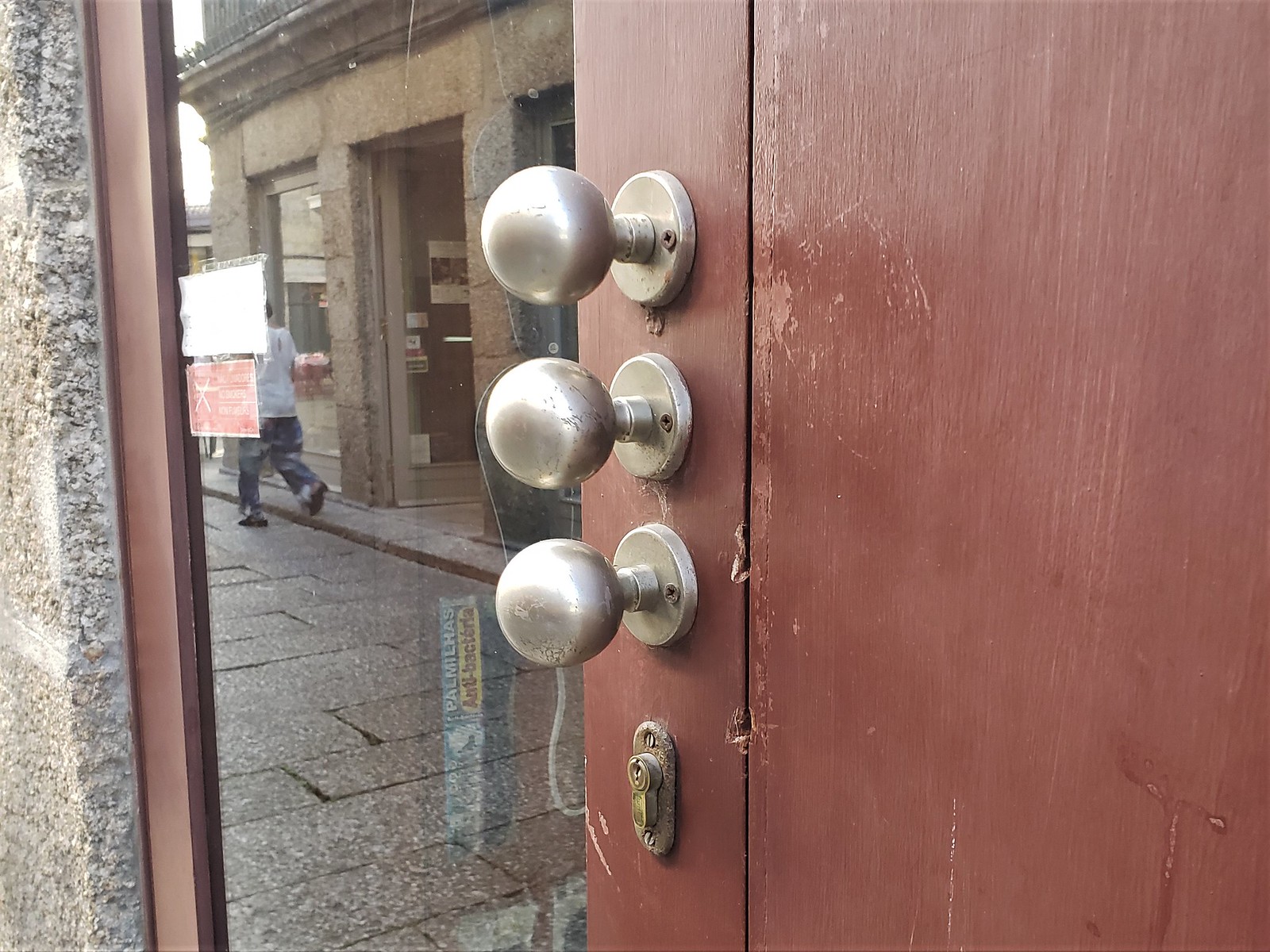This photograph, taken outdoors, captures a unique entrance to a building characterized by a distinct door with three vertically aligned, round doorknobs made of soft, matte-finished silver metal that resembles light bulbs. These doorknobs are identical and each is mounted on a round metal base. Beneath the lowest doorknob, there is an ornate brass keyhole. The door itself is a wooden structure painted in a burgundy color with a blend of brown and red hues. It features a large glass pane that occupies most of its surface, reflecting parts of the surrounding environment including a stone-gray building, a sidewalk made of stone bricks, and the faint silhouette of a person in a white t-shirt and blue jeans, partially obscured by stickers on the glass. The left edge of the image reveals a stone or concrete wall, adding to the outdoor ambiance of the scene.